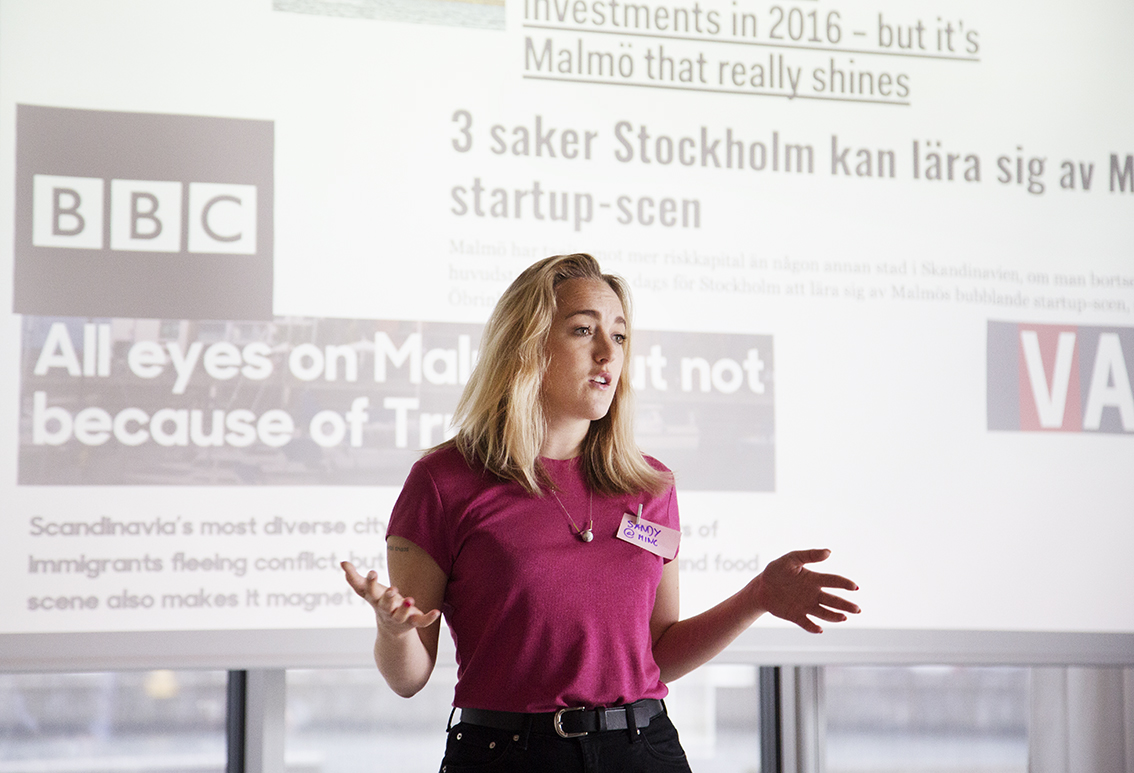The image depicts a woman named Sammy giving a presentation in front of a projector screen filled with various pieces of information and logos, predominantly related to Sweden and Swedish cities. Sammy is wearing a pink blouse with short sleeves, paired with black jeans and a black belt. She has shoulder-length blonde hair and a necklace with a central pendant. A handwritten name tag is pinned to the left side of her blouse. Sammy appears to be in the midst of speaking, with both arms raised as she gestures. Behind her, the projected content includes text such as "Investments in 2016," "Malmo that really shines," and references to "Stockholm," "Kahn," "Lahar," "SIGA," and "Startup CEN." The BBC logo is also prominently displayed. Although the exact details of the text are partially obscured by Sammy, it mentions topics like Scandinavia's diversity, immigrants fleeing conflict, and other economic or social matters, indicating the presentation's focus on regional investments and demographics.